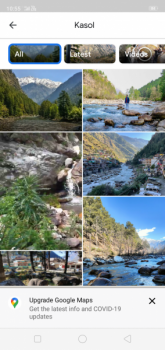The image features a gray border at the top with the text "K-Sol" and an arrow pointing to the left. Below the header, there are three labeled boxes with the text "All," "Latest," and "Video." The "All" section is highlighted and bordered in blue. Beneath these options, there are two columns of three pictures each, with the bottom image in the left column partially cropped out.

In the left column:
1. The top image depicts a serene scene of a stream with surrounding trees and a mountain in the background.
2. The middle image showcases a waterfall cascading over rocks with plants growing along the sides.
3. The bottom image is partially cropped, rendering its content largely obscure and indiscernible.

In the right column:
1. The top image features a person standing on a rock in the middle of a stream, flanked by two large hills on either side.
2. The middle image captures an aerial view looking down at a sprawling valley.
3. The bottom image displays another stream with several rocks protruding from the water.